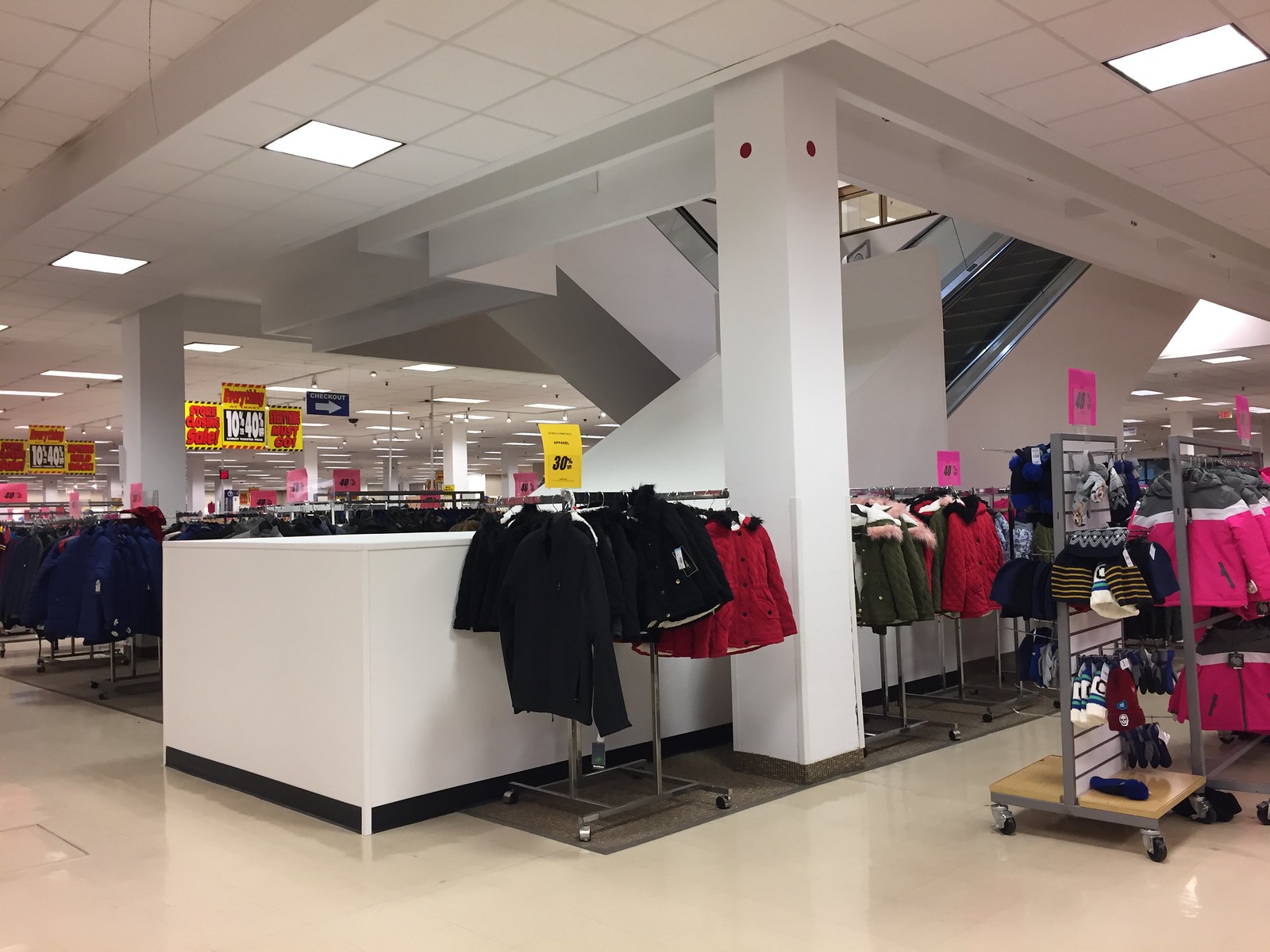The image captures a scene inside a department store reminiscent of classic mall mainstays like Macy's or Dillard's. Centered around an escalator area, both the up and down escalators are prominently visible. The store is brightly lit, emphasizing a vast array of clothing racks spread across the floor. Each rack is adorned with signs promoting a significant sale, with discounts ranging from 10% to 40% off. 

In the foreground, a rack of winter sweaters is clearly marked with a "30% off" sign. Additional pink signs highlight other promotions but their details are less legible. The background reveals more racks, primarily showcasing winter apparel. The overall ambiance of the image evokes a sense of nostalgia, reminiscent of bustling malls in their prime days, filled with enthusiastic shoppers and seasonal deals.